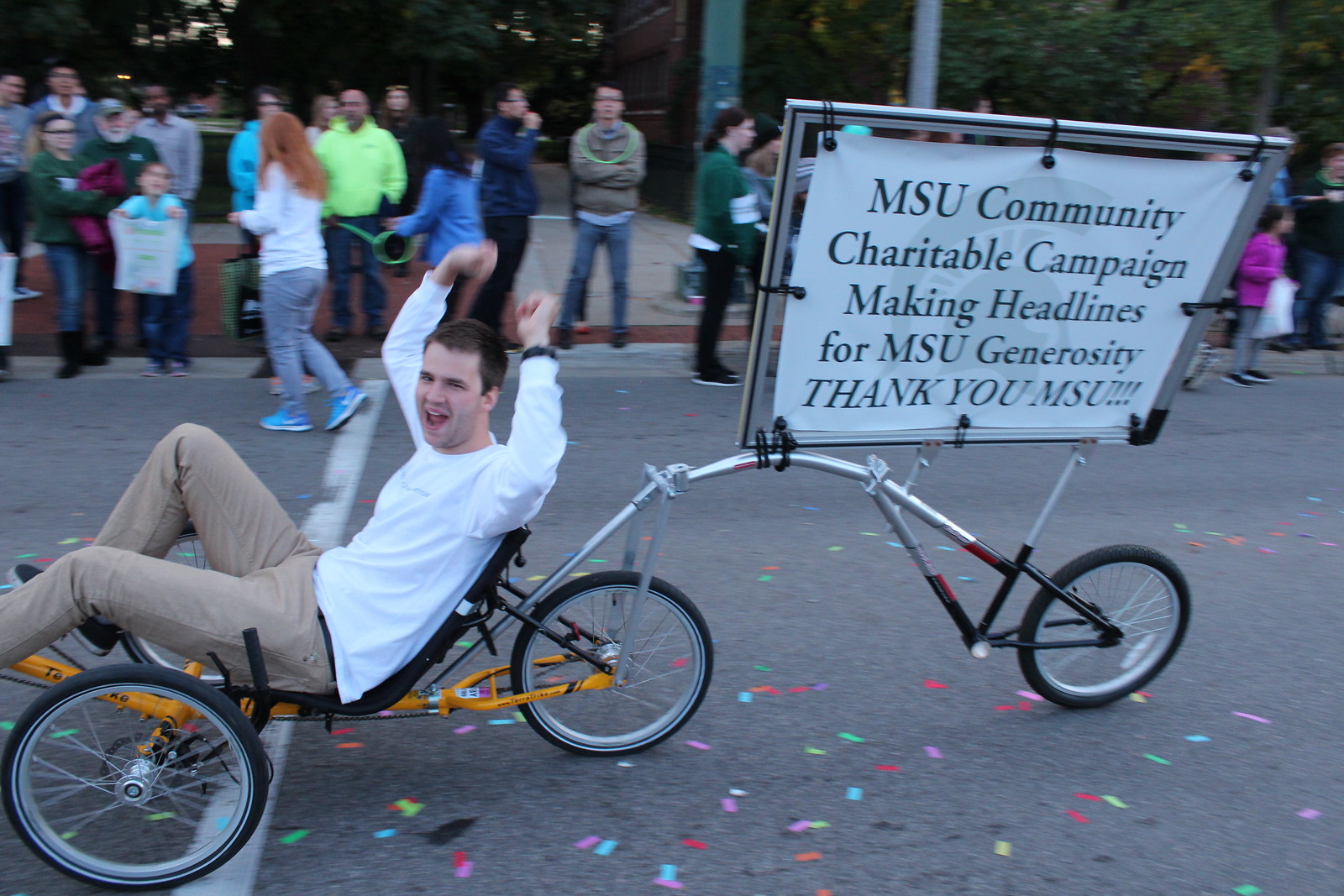This outdoor photograph captures a dynamic scene featuring a man riding a uniquely designed four-wheeled bicycle on an asphalt road, during what appears to be a charity event, indicated by the colorful confetti scattered on the pavement. The man is centrally positioned in the image, and it's a bright, clear day with sky visible in the background. He is dressed in a white long-sleeved shirt and brown pants, shouting joyfully with his hands raised above his head. This unconventional bicycle has a distinctive layout with a wheel at the front, a wheel in the middle, and two wheels at the back. The man is comfortably seated with his back resting against a black seat, his feet extended forward. Behind him, attached to the bicycle, is a prominently displayed poster that reads, "MSU Community Charitable Campaign Making Headlines for MSU Generosity. Thank you, MSU." On the right-hand side of the road, several people are gathered on the sidewalk, observing the event. Further in the background, the scene is framed by bushes, trees, and a lamp post. The photograph bursts with a multitude of colors including shades of gray, red, pink, purple, light blue, dark blue, black, silver, tan, brown, and orange, which contribute to the lively atmosphere of the event.